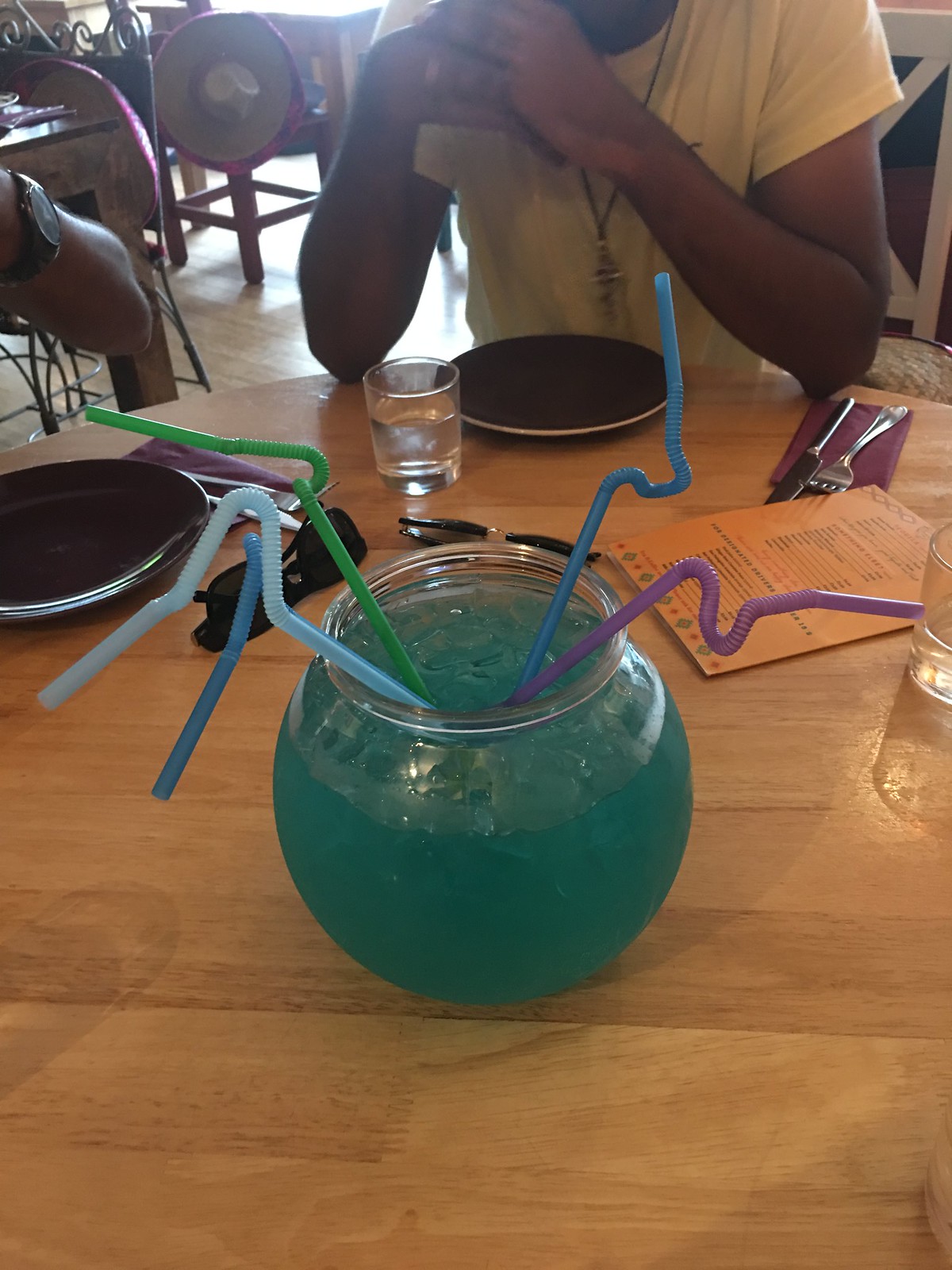This photograph captures a vibrant scene at a restaurant, focusing on a large, round, blonde wooden table made of slats. Central to the image is a sizeable fishbowl-like glass container filled with a turquoise-blue liquid and numerous ice cubes. The fishbowl features five colorful, noticeably bendy straws in shades of purple, blue, light blue, dark blue, and green.

Seated at the back of the table is a dark-complected man wearing a yellow T-shirt and a necklace with a silver ornament on a black cord. He is accompanied by another person to the left, identifiable by their arm and a black watch. In front of the man, there is a black plate with silver rims, a clear short glass, and utensils placed on a purple napkin. The table also holds two pairs of dark-lensed sunglasses, an orange menu, and additional glass cups set upside down to the right.

In the background, one can observe the dining area filled with chair and human legs, adding depth to the lively restaurant atmosphere.